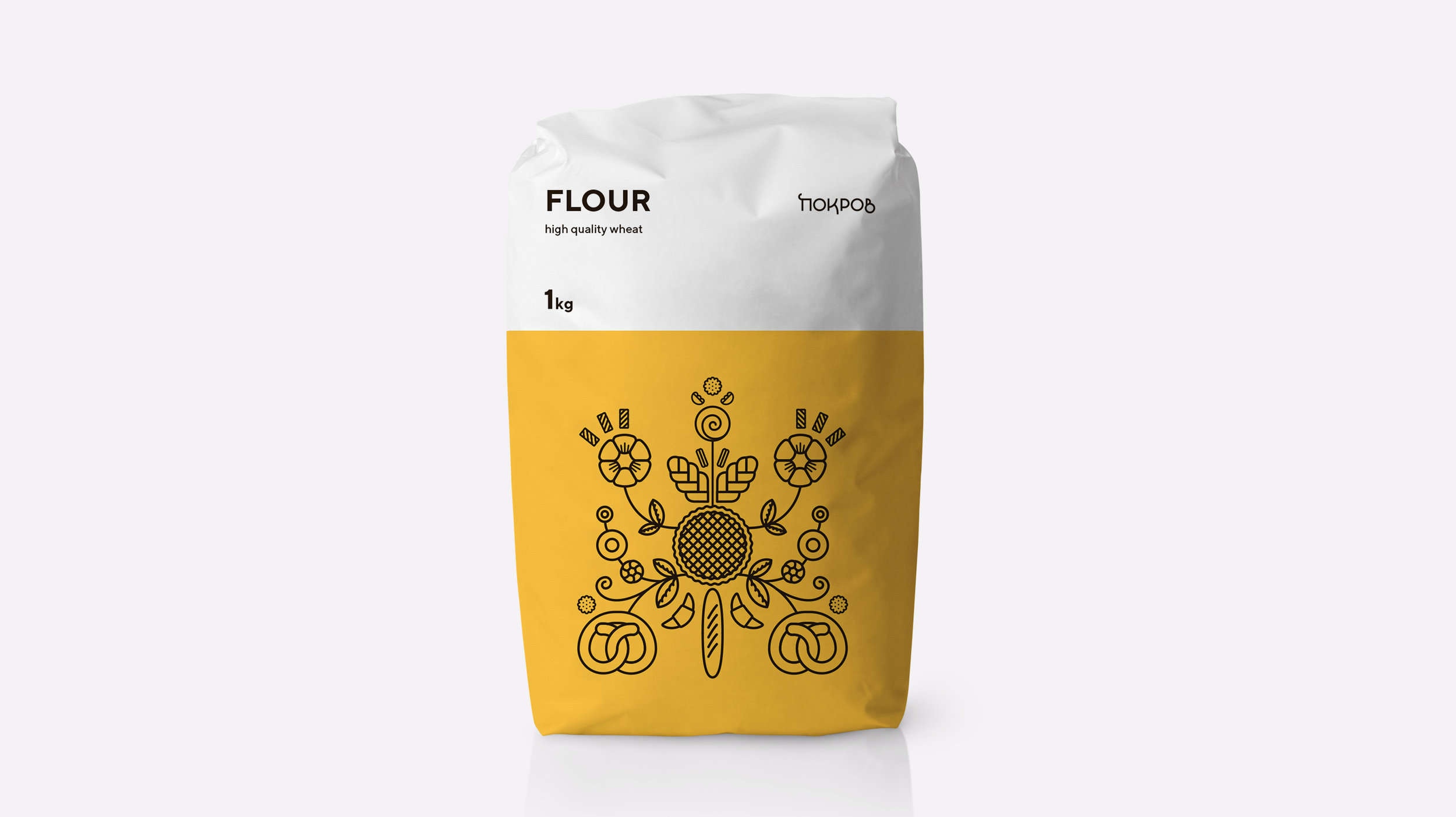This photograph showcases a 1 kg bag of flour prominently displayed against a plain white background. The bag itself is visually divided into two sections: the upper portion is white, while the lower portion features a muted mustard-yellow background adorned with a folk-style illustration. In bold black text at the top of the bag, the word "Flour" is prominently displayed, followed by "high quality wheat" in smaller letters underneath. Below this, the weight "one kilogram" is clearly indicated. The yellow section of the bag is decorated with a medium black line illustration that includes various bread items such as pretzels, bagels, croissants, and pies, interspersed with artistic elements like leaves, flower heads, stems, and spirals, all evoking a sense of home baking. In the top right corner of the bag, there is a logo in a foreign alphabet, adding an additional element of interest. The bag of flour is a crisp, paper type commonly found in grocery stores, folded over at the top to keep it sealed.